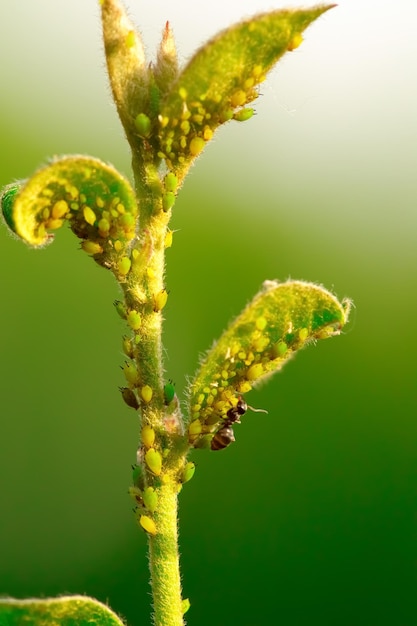This detailed photograph captures a vividly textured plant, prominently centered in the frame. The plant, with a distinct yellow-green hue, is characterized by its fuzzy, fur-like stems and leaves, which bear a resemblance to the texture of a tennis ball. Two pointy stems jut out from the top of the main plant, one extending to the left and another to the right, each covered in tiny bead-like specks in shades of yellow and green. The plant surface is home to an array of small green aphids dotting the leaves and stems. Alongside these numerous aphids, a single black insect, possibly an ant or bee, can be seen on a stem veering to the right. The background of the image transitions from a deep green at the bottom to a light green and finally to an almost white hue at the top, highlighting the plant's vibrant colors and intricate details.